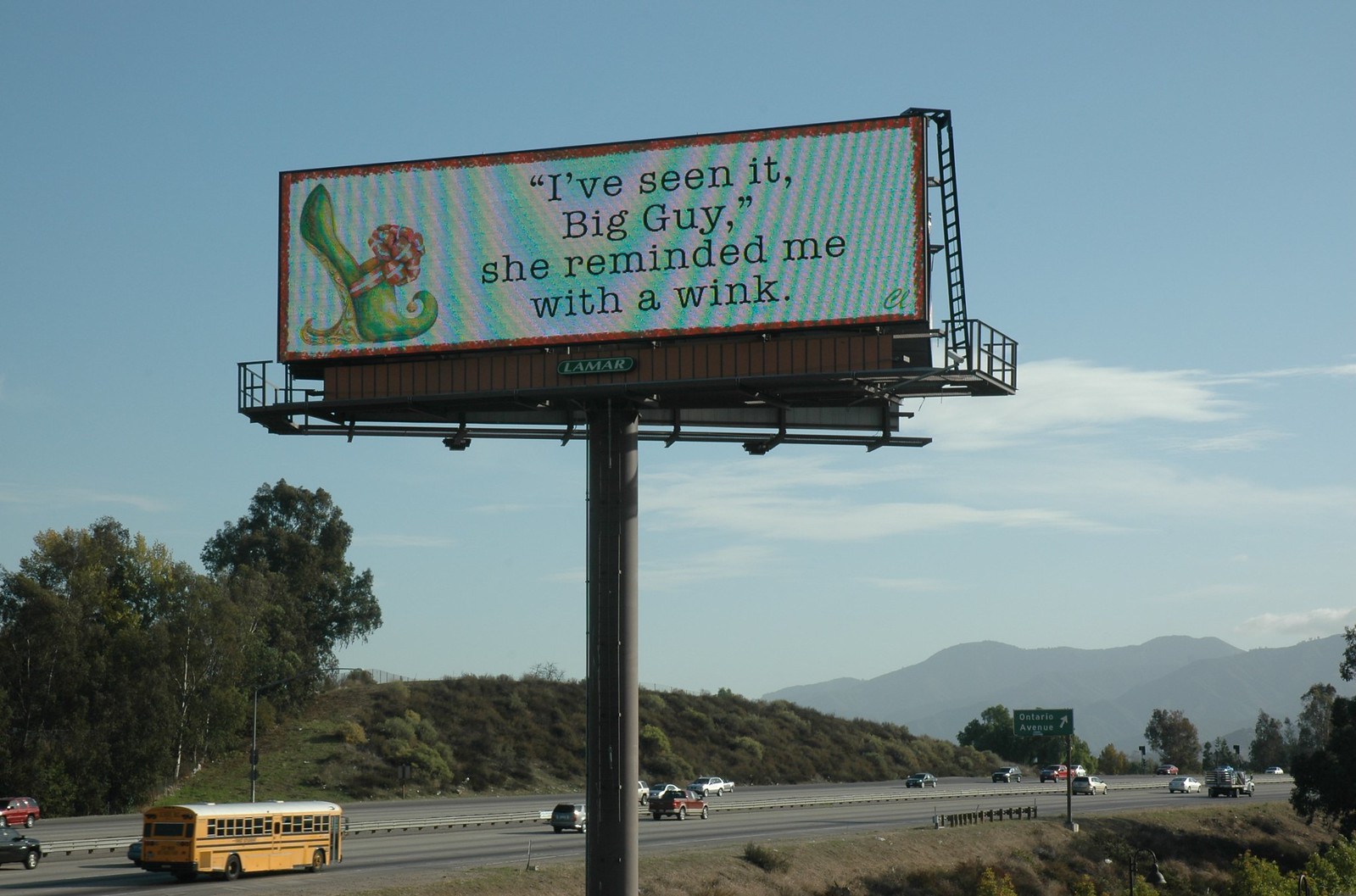In this photograph taken outdoors, we see a wide highway or expressway with a guardrail dividing the opposing lanes of traffic. Several vehicles, including a large yellow school bus, can be observed traveling in both directions. Beyond the road lies a hill adorned with bushes and trees, further stretching into a scenery of distant mountains. Prominently closer to the camera is a billboard that reads, "I've seen it big guy, she reminded me, with a wink." The significance of the billboard's message is unclear, but it may be interpreted as having a Christmas theme.